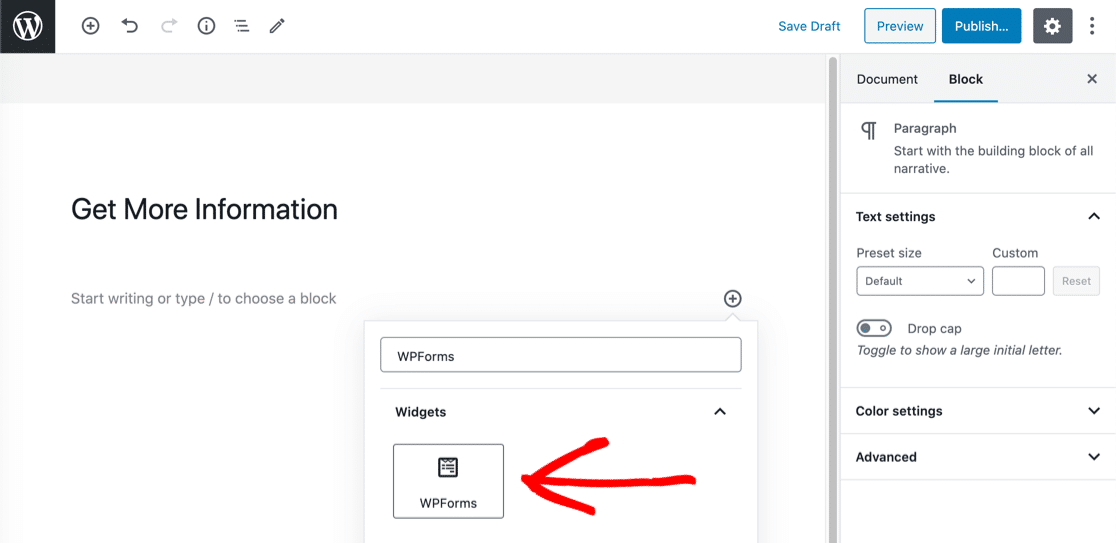The image depicts a WordPress editor interface with various UI elements illuminated. Starting from the top left, there's a prominent "W" icon indicative of WordPress. Below this icon, on the left-hand side, is a section labeled "Get more information." 

Directly underneath, in smaller print and creating a slight gap, it reads "Start writing or type / to choose a block." Progressing downward, the next section highlights "WPForms" followed by a "Widgets" label. A notable red arrow points to a box containing "WPForms," drawing attention to this feature.

At the top of the interface, there are options labeled "Save Draft," "Preview," and "Publish," with the latter button highlighted in a blue box reading "Publish...". Adjacent to these controls, there is a graphical element—a stylized white flower situated within a gray box.

To the right, tabs labeled "Document" and "Block" are visible, with the "Block" tab underscored by a blue line, indicating it is currently selected. Within this tab, the "Paragraph" option is displayed, alongside a symbol resembling a backward letter "P" (¶ icon). Scattered throughout the rest of the interface are additional clickable regions and fillable sections designed for user interaction and content creation.